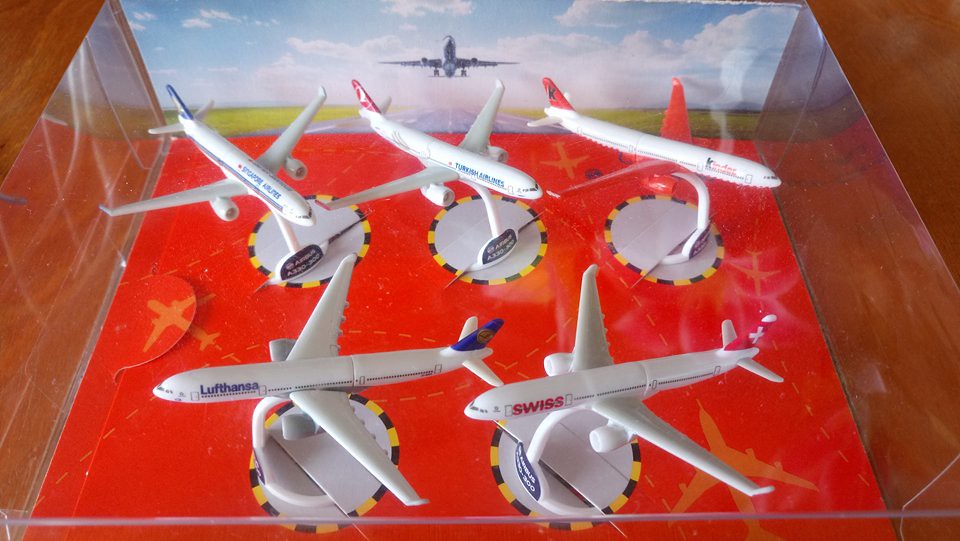This is a color photograph of a display case on a brown wooden table, showcasing five model jumbo jet airplanes. The rectangular, seamless display case, constructed from lucite panels, is oriented in a landscape view. The bottom of the case is covered with a red base featuring gold silhouettes of airplanes and flight patterns. Each model airplane is mounted on a stand that connects to a circular white base with alternating yellow and black markings along its edge.

In the front, the model on the left bears the livery of Lufthansa in blue, while the one on the right displays the Swiss logo in red. The three model planes in the back are smaller and out of focus, making their liveries difficult to read, but there are hints that they might represent Turkish Airlines and possibly Singapore Airlines.

The backdrop inside the case is a paper display depicting a green grass landscape at the bottom third and a blue sky with white clouds for the upper two-thirds. Dominating the background is an image of a real jumbo jet ascending at a 45-degree angle, enhancing the overall aviation theme. The detailed elements of the models and the background create a cohesive and engaging display for aviation enthusiasts.